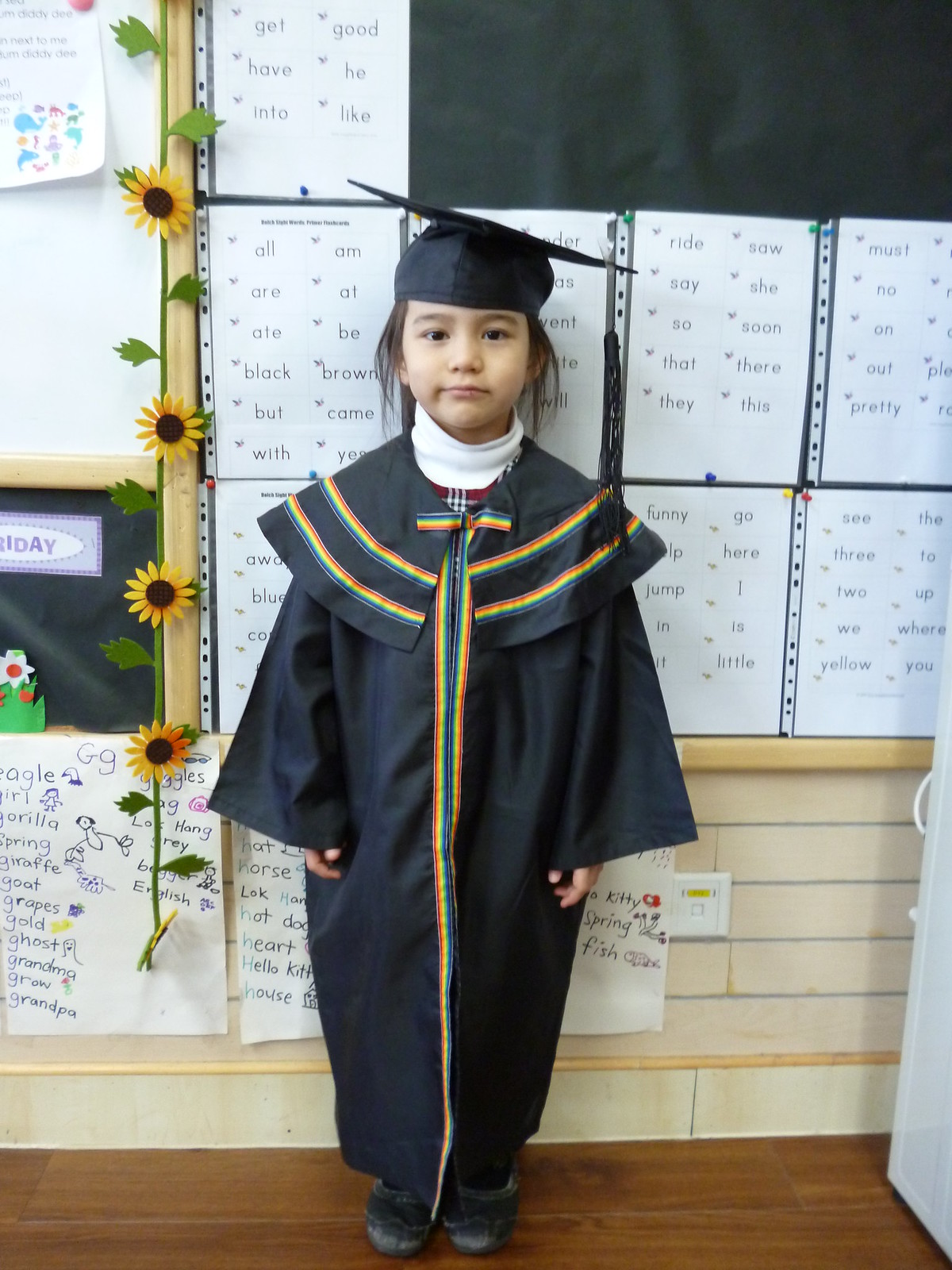The image captures a young girl, approximately first-grade age, donned in a graduation cap and gown. The cap is a black mortarboard, slightly tilted to one side, and the black gown features vibrant rainbow-colored ribbon and arcing lines along the front seams and collar. Beneath the gown, she is wearing a white turtleneck and black slippers. She stands on a brown, hardwood floor in what appears to be a classroom. Behind her is a blackboard adorned with various student-made projects and white papers with single words, likely for learning purposes, pinned to it. To her left is a bulletin board decorated with four sunflowers, possibly plastic, connected with a green string. A white cabinet and more pinned papers are visible in the lower right corner. The upper part of the photograph has a noticeable black space. The scene is completed with a glimpse of a white wall with blue lines further enhancing the classroom setting.